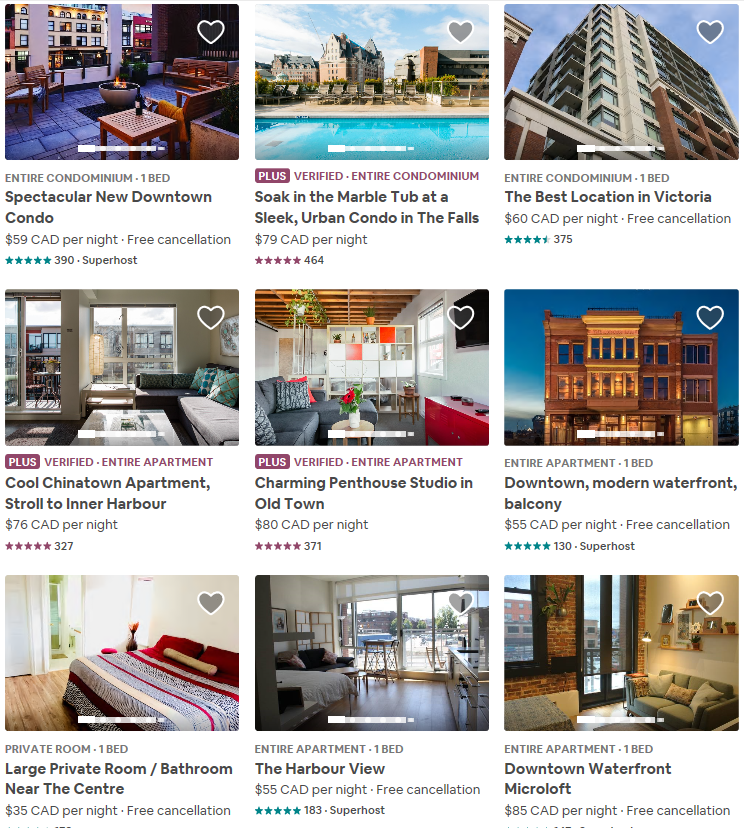Caption:  
A screenshot displaying a section of my website featuring a grid layout of hotel listings. The grid is organized with three hotels per row, presenting a total of nine listings. Each hotel entry includes a captivating image of the property, with a heart icon positioned at the top right corner for users to save their favorite options. Below the image, the type of stay is highlighted and followed by a brief description. The nightly price in CAD is prominently displayed beneath the description. Additionally, there's a star rating system using either blue or purple stars to represent guest reviews.

The first hotel listing showcases an entire condominium with one bed, titled "Spectacular New Downtown Condo," priced at 59 CAD per night. It features three five-star ratings and includes a note indicating it's a "plus verified entire condominium." Another entry highlights a "Marble Tub at a Sleep Urban Condo in the Falls," available for 79 CAD per night.